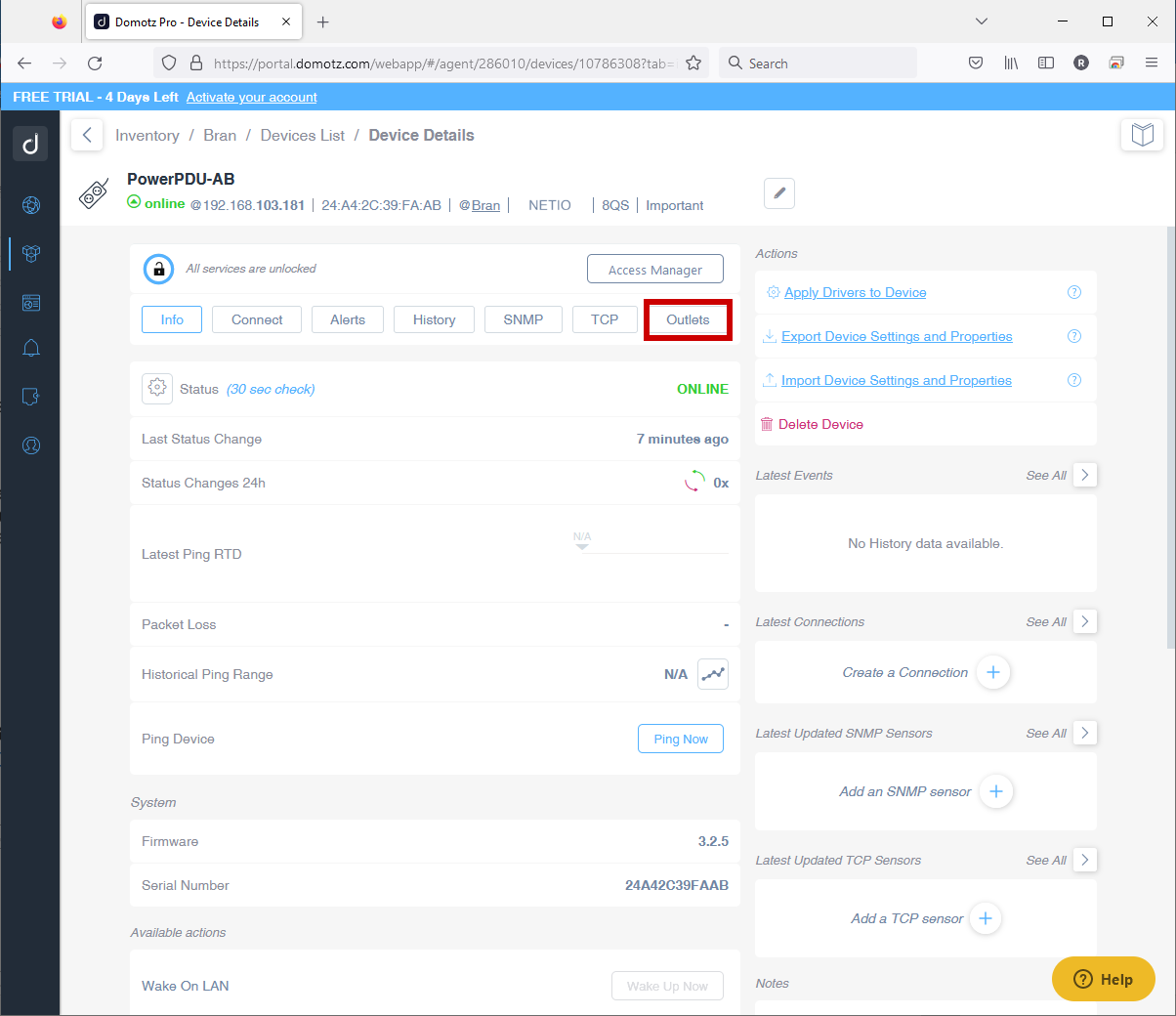This image is a screenshot from a web page displaying detailed information about the "Doughnuts Pro" device. At the top, a light royal blue rectangle spans the width of the page, prominently featuring a countdown saying, "Free trial - 4 days left," and a call to action, "Activate your account." 

The left sidebar is black, adorned with various teal-colored icons—six in total—with the topmost icon in white, indicating its selectable status. 

Midway down the page, there’s a section titled "Power PDU - AB," showing the device's status as "online" in green font, with an additional note that says "All services are unlocked." Adjacent to this, an information section is expanded, while other navigation options include "Connect," "Alerts," "History," "SNMP," "TCP," and "Outlets." Notably, the "Outlets" section is highlighted with a red rectangular outline.

Finally, the lower right corner features a yellow help button, ready to assist users with any inquiries. This image captures a comprehensive overview of the device management interface.